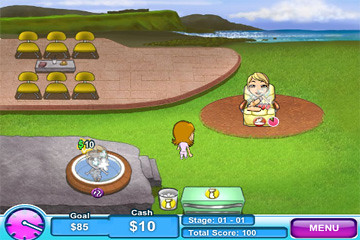The screenshot captures a moment from a mobile or laptop game set within a colorful, virtual environment. At the center, a child character stands on a circular wooden ramp, while another child stands facing her. To the side, there's a small, water-style pool with a child inside, accompanied by a rating of £10. The game's interface reveals that the player currently has $10 in cash, working toward a goal of $85. Positioned in Stage 1 of the game, the player has achieved a total score of 100 points. The setting showcases a verdant grassy area adjacent to a beach, with clear sunny skies and a vast sea stretching into the horizon, hinting at a leisurely, outdoor adventure theme.